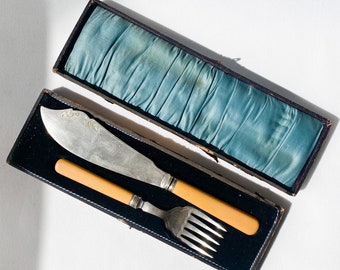The image depicts an old-fashioned utensil set housed in a fabric-lined case. The case's lid is lined with a teal blue or satin-like fabric, while the section holding the utensils is black. The set includes a large, distinctively shaped knife resembling a kukri, and a fork with an unusual five-prong design, contrary to the more typical three or four prongs. Both utensils feature sturdy brown wooden handles, and their metallic parts appear well-used. The background of the image is white with a noticeable shadow to the left, adding depth to the setting. The utensils are positioned at a slanted angle within the case, suggesting an elegant yet functional presentation.